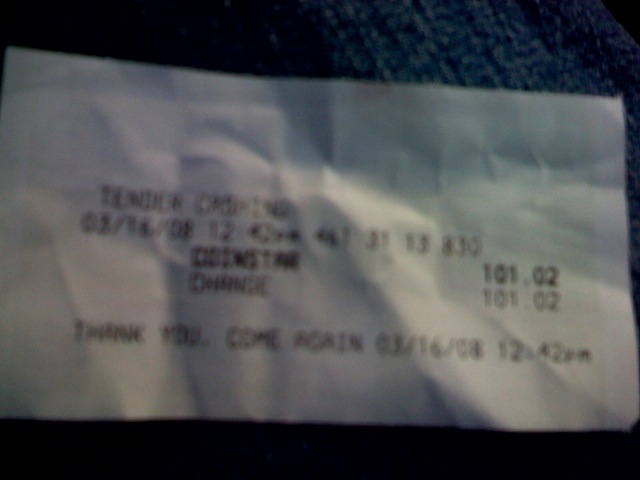In the image, there is a small, rectangular white receipt laying on a predominantly blue background that appears to be fabric, possibly blue jeans, suggested by the visible texture in the upper right corner. The rest of the background is mostly black, making the blue fabric more noticeable. The receipt itself is somewhat wrinkled and appears to have been folded multiple times. The print on the receipt is black and slightly blurry, making it challenging to read, but key details are still discernible. It mentions "Tender ordering" followed by "316.08," with the time stamped as "12:42 p.m." The receipt also lists "Coinstar" next to the amount "101.02" and repeats "Change 101.02." At the bottom, it states, "Thank you. Come again," along with the date "3-16-08" and the time "12:42 p.m."